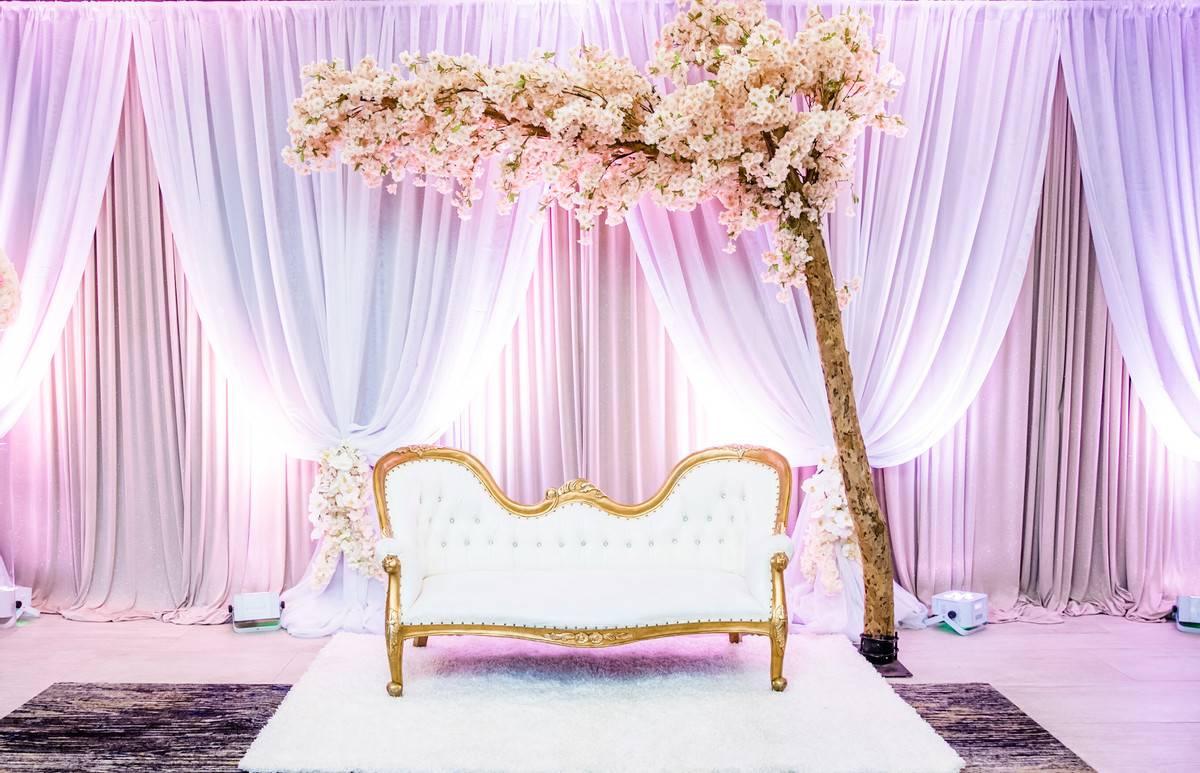This photograph depicts a lavish, ornately detailed room that evokes the elegance of French provincial design. At the center of the scene is a tufted, white loveseat adorned with gold trim, exuding a regal air. The loveseat is positioned atop a layered arrangement of rugs—a fluffy white throw rug lies directly beneath it, followed by a dark rose-colored carpet, and finally a lilac-colored rug, all contributing to the room's opulent texture.

Adjacent to the loveseat stands a tall, intriguing tree with a trunk, whose branches are heavily laden with pink and white blossoms, reminiscent of Japanese cherry blossoms or sakura flowers, adding a touch of nature's beauty to the indoor setting.

The backdrop is particularly captivating, featuring floor-length, gauzy curtains in variegated shades of pale pink, lavender, and bluish-purple, gathered with bunches of flowers. These draperies are lit dramatically by strategic floor lights, enhancing their ethereal quality and creating a stunning visual contrast.

An additional object, which appears to be a white plastic picnic basket or cooler, is subtly placed in the background, hinting at a whimsical or theatrical element within the décor. The overall scene exudes an air of luxury and fantasy, reminiscent of an elegant dressing room, a dramatic play setting, or a meticulously curated photo opportunity area, potentially for a wedding or similar celebratory event.